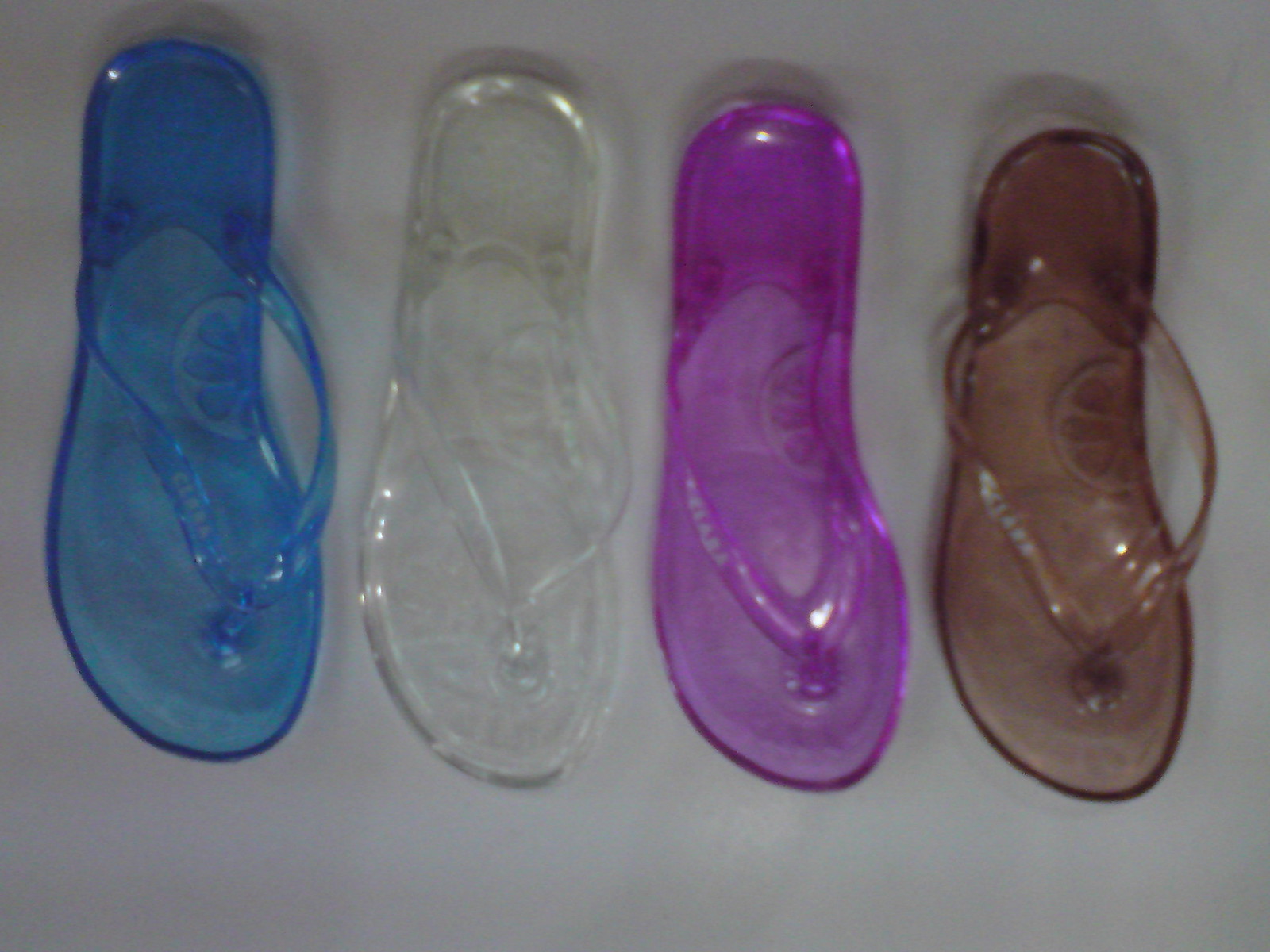This color photograph features four jelly flip-flops, placed on a gray surface. Made from a clear, see-through material akin to that used for Crocs, these flip-flops exhibit varying degrees of translucency, allowing for objects beneath to remain visible. In sequence from left to right, the colors are vibrant purple, clear white, lavender, and smoky brown. A distinguishing feature of each flip-flop is a half citrus fruit slice – matching the flip-flop’s color – embedded at the arch. The background showcases subtle shadows cast by the flip-flops, suggesting a light source outside the frame. The flip-flops exude a playful, summery vibe, possibly intended for poolside use. The image is slightly out of focus, enhancing the ethereal quality of the translucent footwear.